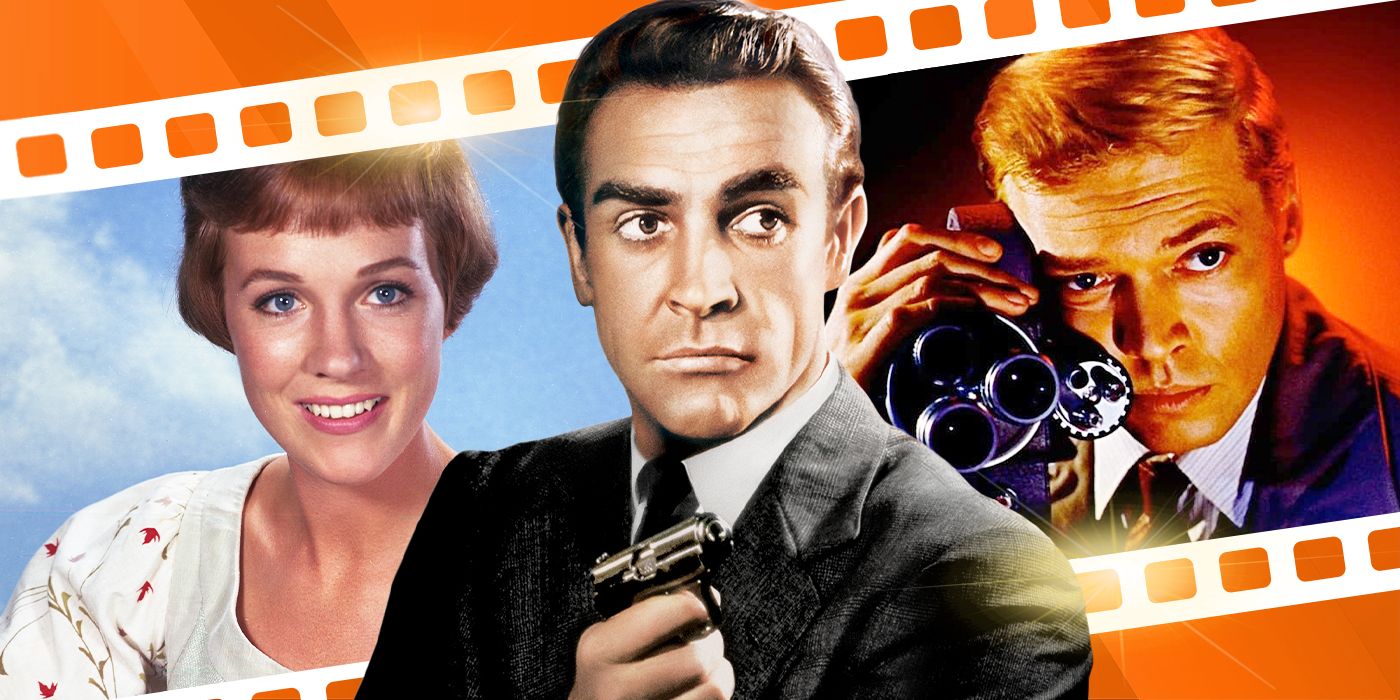The movie poster features three iconic figures from the cinematic world, depicted in a film strip motif with distinct backgrounds. On the left stands Julie Andrews, wearing a white shirt with a subtle print and smiling against a blue sky backdrop. In the center, Sean Connery embodies his classic 007 persona, holding a pistol in his right hand, dressed in a suit jacket, white buttoned-up shirt, and black tie. His dark hair and eyebrows contrast against the background which includes black and orange hues. On the right, a man with blondish auburn hair is captured holding a three-lensed camera, dressed in a blue suit jacket, maroon tie, and striped white shirt, set against an orange background with dark shadows. All three figures are Caucasian, with the central image of Connery superimposed prominently over the film strip design.